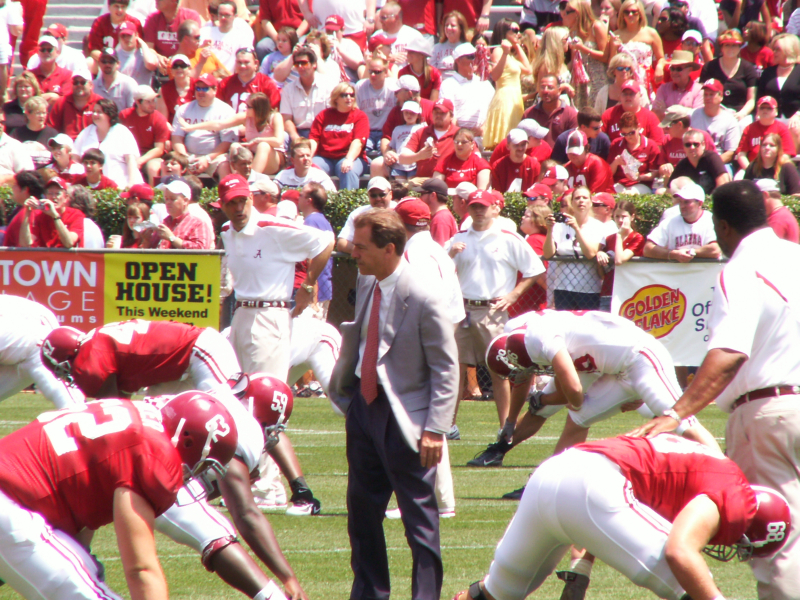The image depicts Nick Saban, the coach of the Alabama Crimson Tide college football team, during a practice session outside on a sunny day. Saban stands prominently in the center of the field, dressed in a gray suit, red tie, and white collared shirt, with black khakis. Surrounding him are multiple football players wearing red and white jerseys with matching white tights, engaged in stretching exercises. You can also see Alabama assistants in the area, easily identified by their white polo shirts with red accents. The green grass field is bright under the sunlight, and the background reveals a bustling crowd in the stands, primarily dressed in red and white attire. Behind a row of green shrubbery at the edge of the field, fans stand behind a fence adorned with advertising banners, including messages like "Open House This Weekend" and "Golden Flake." The scene captures a lively and organized moment of preparation before a game.